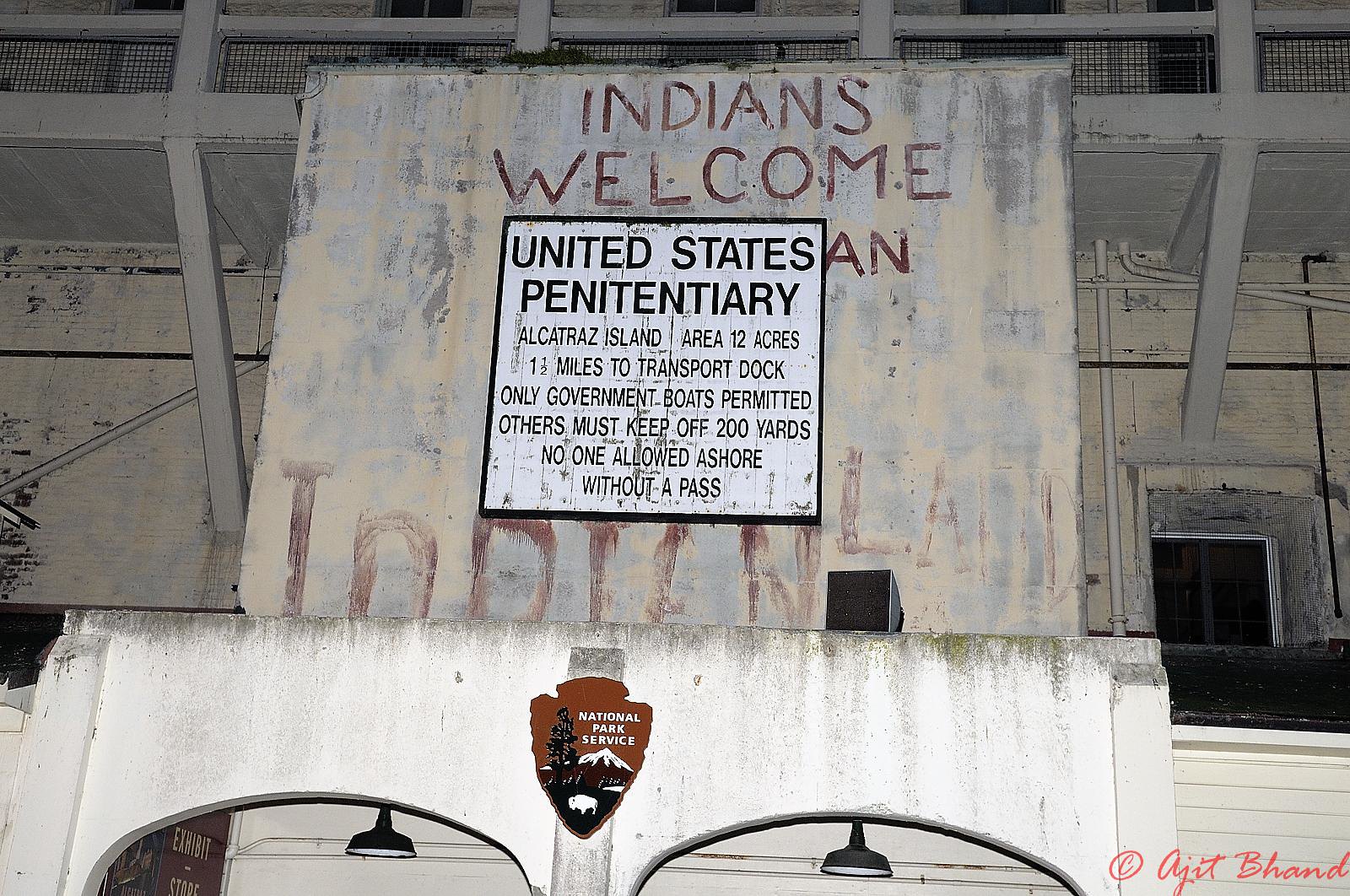The photograph captures the exterior of an old, weathered building, most likely on Alcatraz Island, reflecting its historical significance as a former penitentiary and its current status as a National Park. The building's facade, which appears to be a stone wall with aged, worn paint, displays multiple signs and intricate details. At the top, a partially visible bold red inscription reads "Indians Welcome," with "Indian land" below it. This graffiti-like text appears hand-painted and contrasts with the more formally presented sign beneath it.

The more prominent sign, bordered in black, features neat black script on a white background, detailing specific information: "United States Penitentiary, Alcatraz Island, area 12 acres, 1.5 miles to transport dock, only government boats permitted, others must keep off, 200 yards, no one allowed ashore without a pass." Below this main sign, there's another smaller brown sign featuring the National Park Service logo, depicting a snowy mountain, a white ship, and a tree, reinforcing the site's protected status.

Other elements in the scene add to the historical and slightly decayed charm: lamps hang down from an archway beneath the signs, a black speaker is mounted above, and there are intricate details like black piping, railings, and possible fungus growth on the walls. A white walkway with a small fence leads up towards the building, indicating an entrance. The bottom right of the image bears the copyright name "Ajit Bandh," attesting to the image's authenticity.